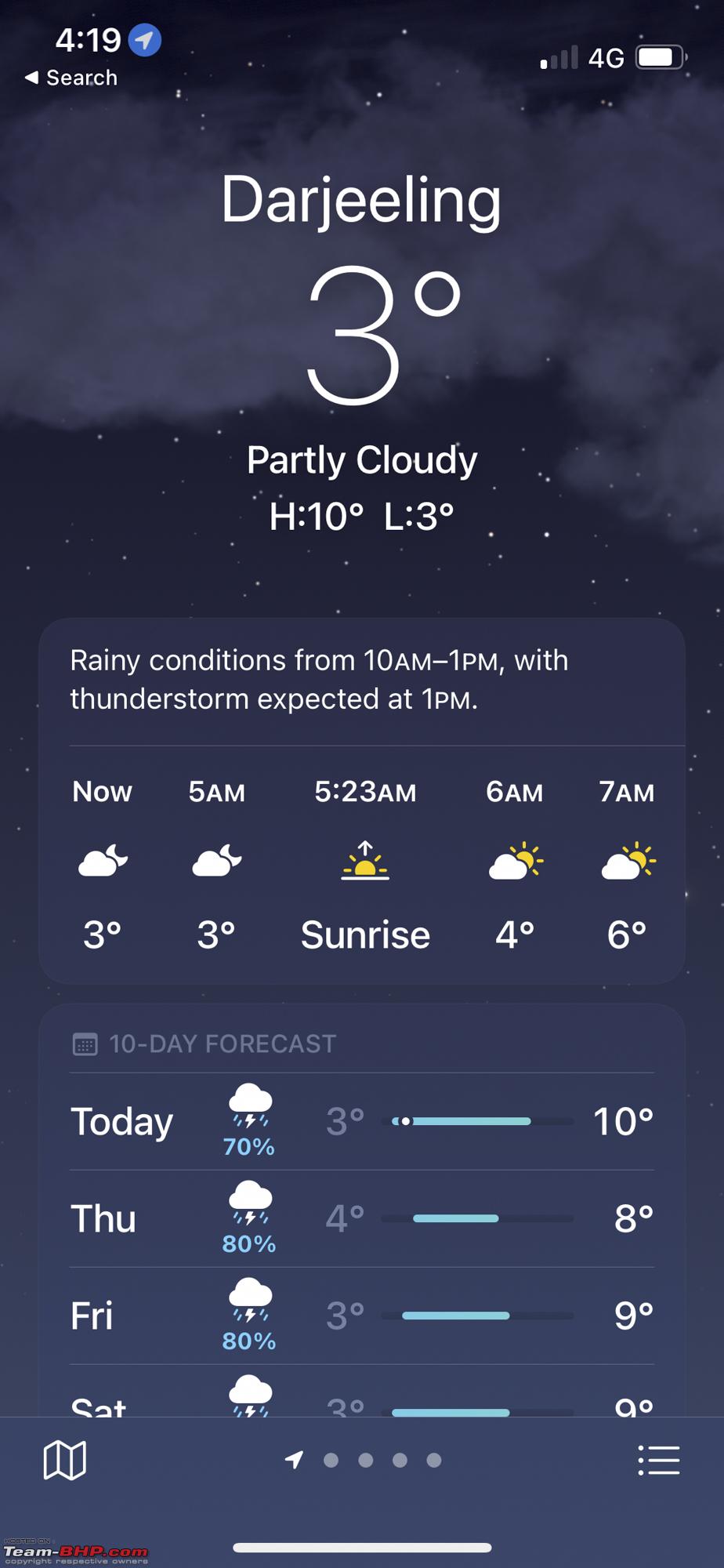A detailed screenshot of a weather app displayed on a smartphone. The status bar indicates the screenshot was taken at 4:19 with a 4G connection and the battery at around 90% charge. The app has a night scene background featuring a very dark blue sky dotted with white stars and dark gray clouds.

At the top, the weather for "Darjeeling" is displayed, showing a current temperature of 3°F. Below the location and temperature, it states "Partly Cloudy" with a high of 10°F and a low of 3°F. It also notes that there will be "raining conditions from 10 a.m. to 1 p.m. with thunderstorms expected at 1 p.m."

The day's forecast chart spans from the current time ("Now") to 7 a.m., providing a three-hour forecast. Below this is a condensed 10-day outlook, currently showing four days: "Today," "Thursday," "Friday," and "Saturday."